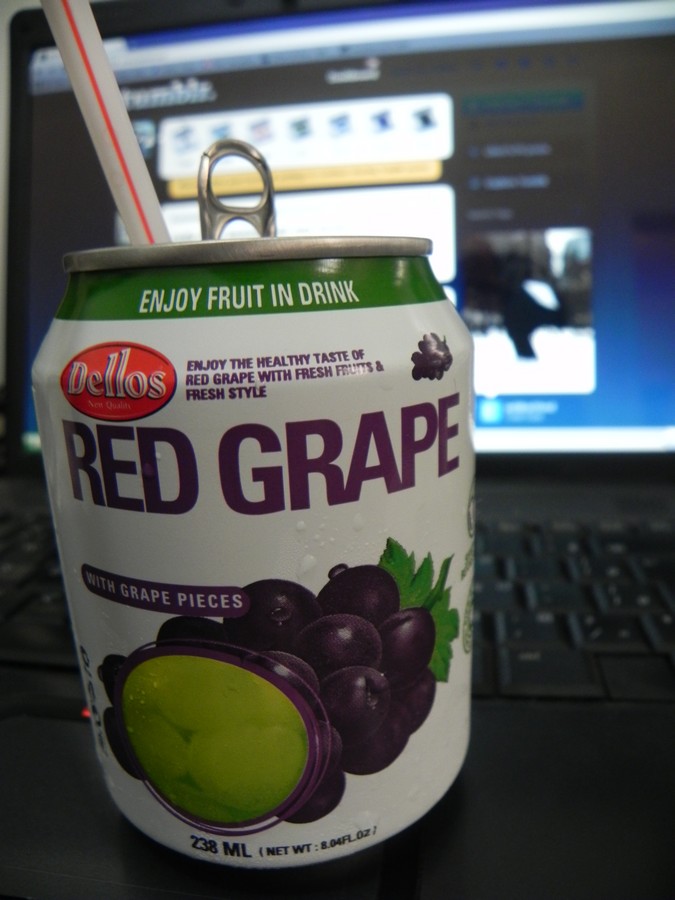The image shows an aluminum can of Delos red grape juice resting on an open laptop, with the can being the focal point. The can has a white background and features an orange oval with the brand name "Delos" displayed in white text. Above this, a red bar with white text says, "Enjoy fruit and drink," and below it, in black font, the tagline reads, "Enjoy the healthy taste of red grape with fresh fruits and fresh style." Further down, the text "red grape" is written in purple, followed by an indication that the juice contains grape pieces. The can displays images of purple grapes alongside a green fruit that is not clearly identifiable, possibly a lemon given the yellow spot visible near the grapes. The contents are labeled as 238 milliliters (8.04 fluid ounces). A plastic straw sticks out from the open tab at the top of the can. Behind the can, the laptop is open, showing the keyboard and a screen displaying Tumblr, with some visible images. The laptop appears to be black. The overall setting suggests that the person is enjoying the beverage while seemingly engaged with the laptop.